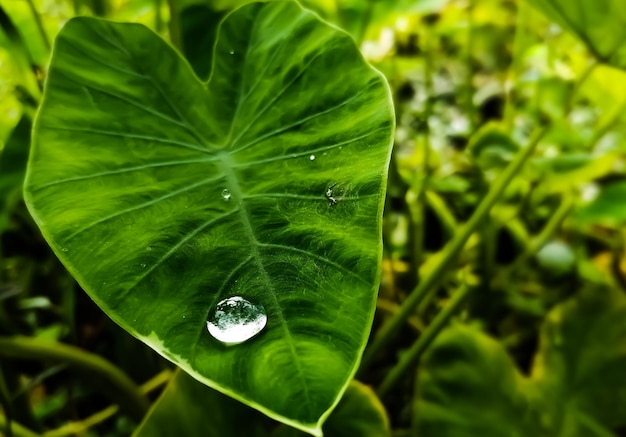This photograph captures a lush, densely vegetated area, resembling a jungle or dense forest. The main focus is a large, heart-shaped green leaf, likely belonging to a philodendron or elephant ear plant. This prominent leaf features thick, veiny lines and is adorned with multiple water droplets. Among them, one particularly large, clear droplet stands out near the edge, reflecting the surrounding greenery. The leaf and its glistening droplets dominate the foreground, while the background is a soft blur of various green plants, stems, and foliage. The overall color palette includes deep greens and light yellowish hues, interspersed with shadows, suggesting a dense canopy that allows limited sunlight to filter through.